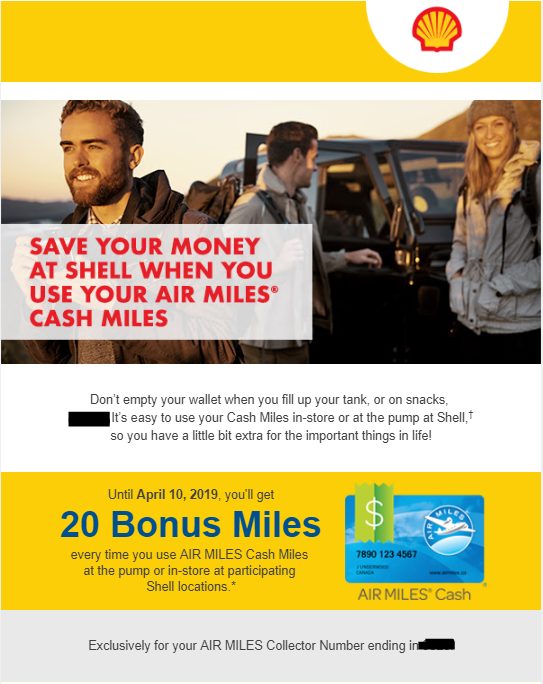A vertically oriented promotional image, likely designed for smartphone and computer screens, features an advertisement for Shell services. 

**Top Section:**
- A yellow rectangular banner spans the top of the image.
- Toward the right of this banner, there is a cutout utilizing the white background, displaying a small Shell logo.

**Main Image:**
- Below the yellow banner, a photograph depicts three young adults (two males and one female) disembarking from a car in a hiking setting. The car doors are open, indicating their recent arrival.

**Promotional Text:**
- A red inset box covers part of one male, with text promoting Shell savings: "Save your money at Shell when you use your Air Miles and Cash Miles."
- Beneath the red box, a white rectangular box encourages: "Don't empty your wallet when you fill up your tank or on snacks."
- Following this, a black box seems to obscure additional information, bearing the message: "It's easy to use your Cash Miles in-store or at the pump at Shell. So you have a little bit extra for the important things in life."

**Offer Details:**
- Another yellow box highlights a special offer: "Until April 10th, 2019, you'll get 20 bonus miles every time you use Air Miles Cash Miles at the pump or in-store at participating Shell locations." 
- It adds a note about exclusivity: "Exclusively for your Air Miles collector number ending in [blacked out]."

**Visual Elements:**
- Embedded within the top yellow section is an image of an Air Miles Cash card, resembling a credit card in blue, accented with a green section featuring a white dollar sign.